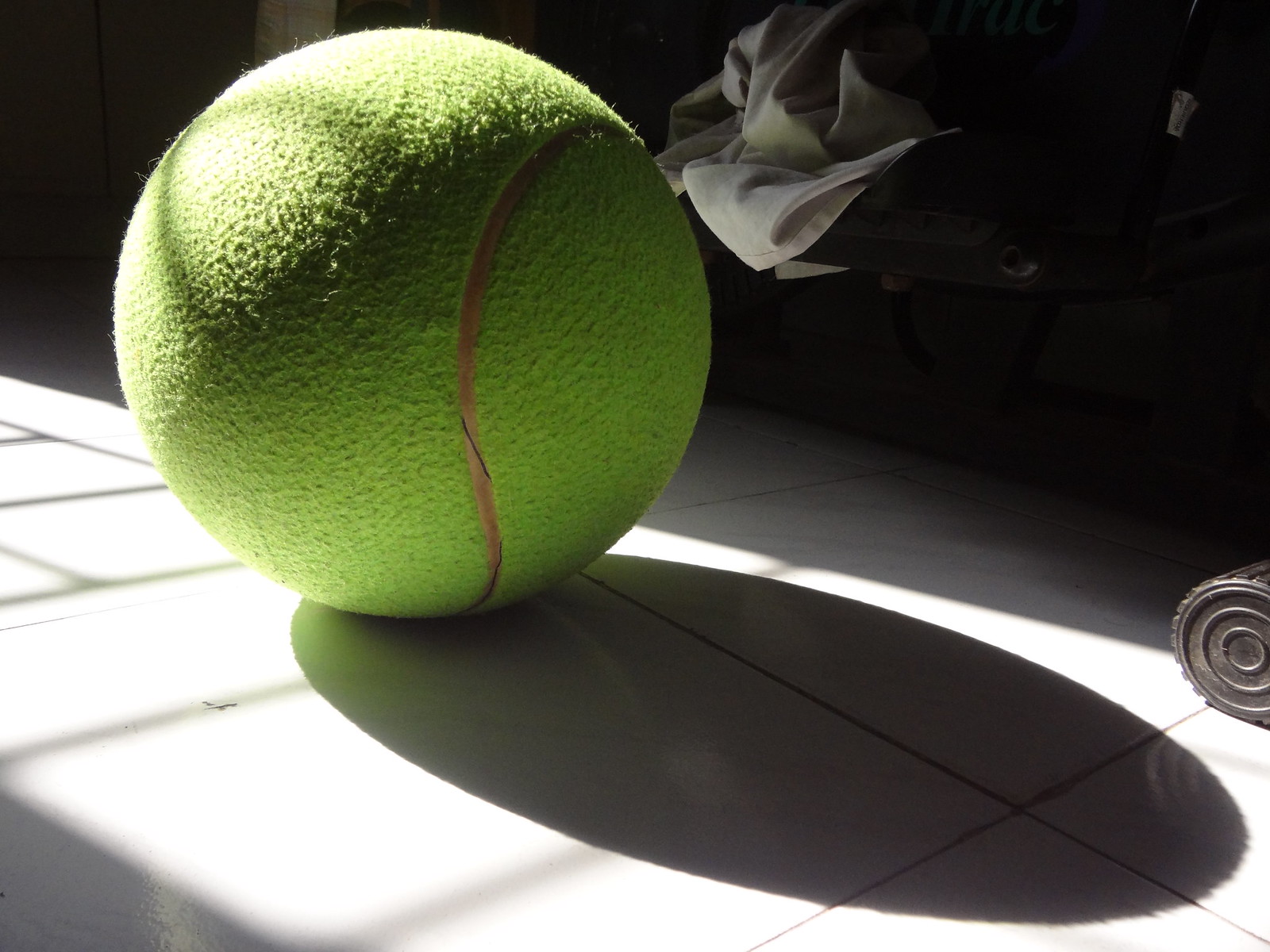In this detailed image, a large, old, lime greenish-yellow tennis ball with a distinctive red stripe along the right side, and a black line running down the seam, is prominently placed on a white tile floor. The tennis ball casts a prominent shadow, indicating a strong light source. To the right of the ball, a white rag is noticeable. Behind the tennis ball, there is a black suitcase with a black handle and a prominent black wheel, suggesting it is used for rolling. The suitcase is partially open, revealing some clothing inside, with a white item of clothing particularly noticeable. There is also partial lettering visible on the suitcase, possibly indicating the brand or logo with "RAC" being discernible. The scene suggests a casual, possibly travel-related setting.